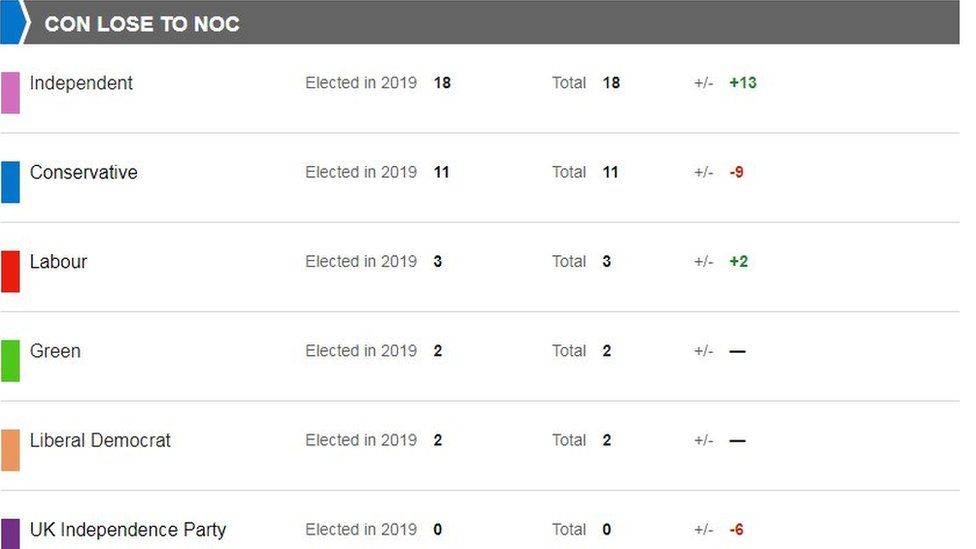A detailed visual representation of election or polling results from 2019 is shown on a white background. The chart features a gray bar at the top labeled "Independent," accompanied by a purple rectangle. Each political party is represented by distinct colors: blue for Conservative, red for Labour, green for Green Party, and coral for Liberal Democrat. The UK Independence Party is also indicated in purple. The results are depicted with numerical values: Conservative with +18 in blue, Labour with -9 in red, Green Party with +2 in green, and Liberal Democrat with a flat line. Additionally, the chart shows Independent at -6 in red. The image illustrates the dynamic shifts in support for each party, reflecting the outcome or sentiment captured during the 2019 elections, with numerical values showcasing gain or decline in support for each party.